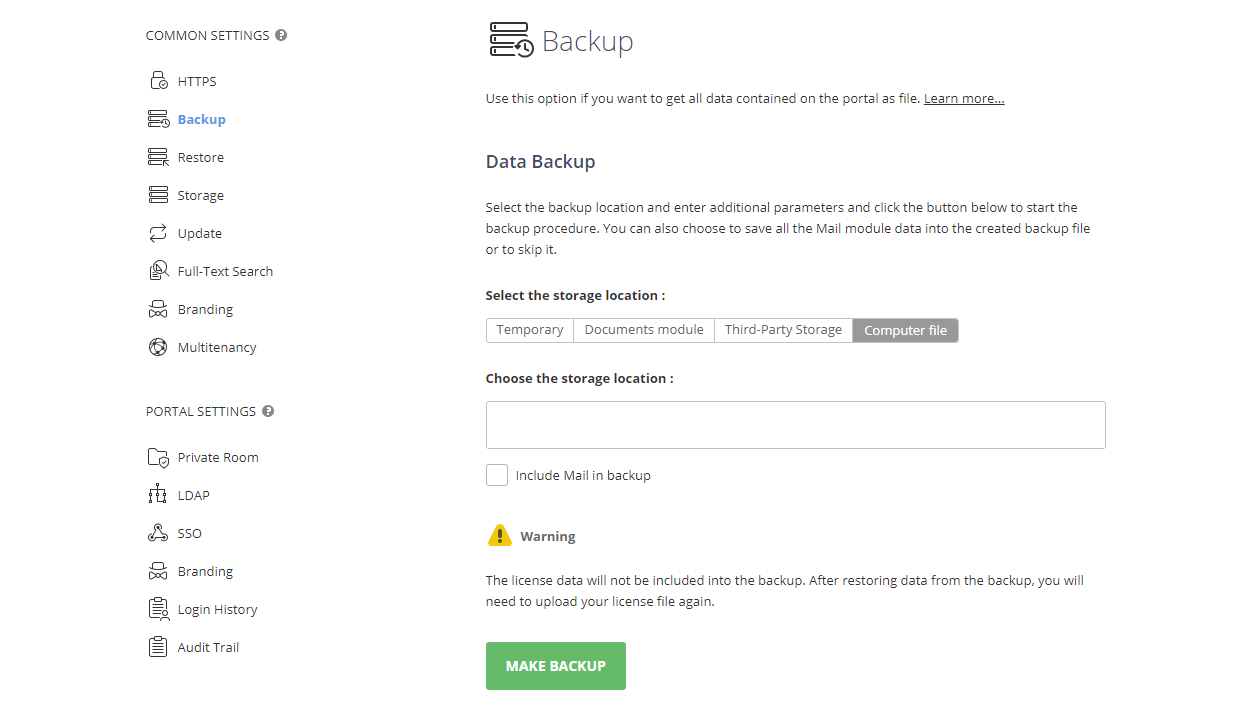**Detailed Caption:**

The image showcases a screenshot of the settings menu, likely from a Windows interface, with a white background. On the left side of the screen, there is a vertical list of clickable settings options under the heading "Common Settings" displayed in black font. The list includes various options such as "HTTPS," "Backup" (which is currently selected and highlighted in blue), "Restore," "Storage," "Update," "Full Text Search," "Branding," and "Multi-tenancy." Below this, there is another heading labeled "Portal Settings" with options like "Private Room," "LDAP," "SSO," "Branding," "Login History," and "Audit Trail."

To the right, the "Backup Settings" page is open. At the top of this page, the word "Backup" appears in black font with an icon to its left depicting three lines and a clock. A brief description underneath reads, "Use this option if you want to get all data contained on the portal as a file," followed by a clickable "Learn More" link. Further down, the section titled "Data Backup" instructs users to "Select the backup location and enter additional parameters and click the button below to start the backup procedure." Additionally, users have the option to include or exclude all mail module data in the backup file. Lastly, the caption mentions the prompt to "Select the storage location" for the backup.